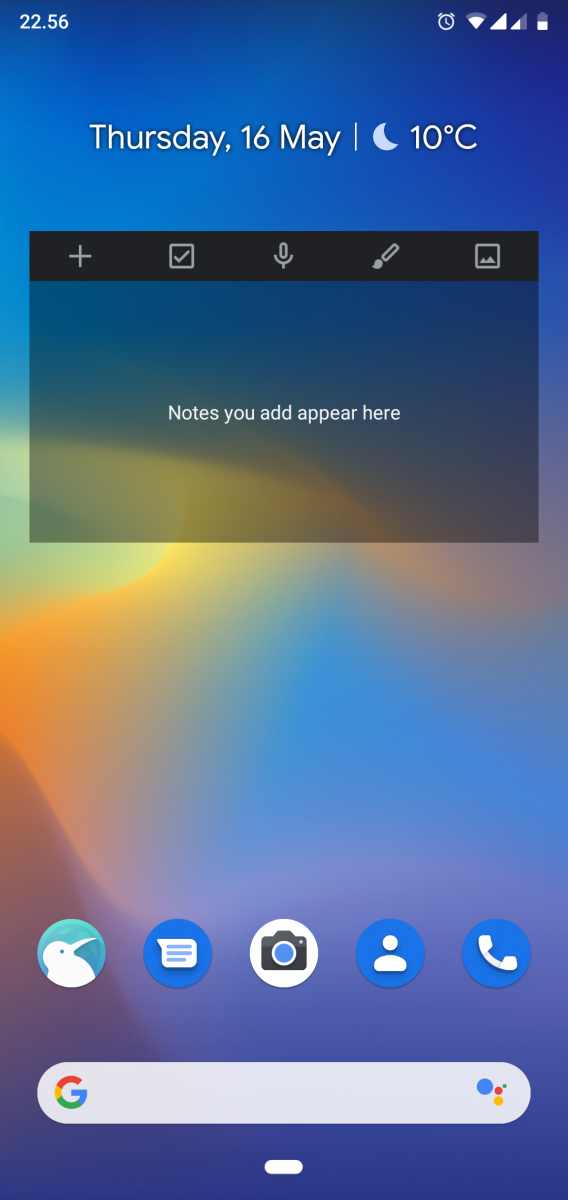The image appears to be a screenshot from an Android device featuring a vibrant, gradient background that transitions through a spectrum of colors: starting from a serene blue at the top, progressing to a bright yellow towards the lower left, shifting into orange and then reddish hues as it moves diagonally to the bottom right, and finally fading back into a darker blue at the very bottom.

In the upper left corner, the time is displayed in a white font as "22:56" (or 10:56 PM). Adjacent to the time, icons indicating the phone’s status are present: a blank space followed by an alarm clock icon, a Wi-Fi signal icon, a mobile signal icon with two bars (one full, one not), and a battery icon showing approximately 50% charge.

At the center of the screen, the current date and weather conditions are shown. It reads "Thursday, 16 May" followed by a small dash. A delicate baby blue crescent moon icon is displayed, accompanied by the temperature "10°C" (10 degrees Celsius).

Below this, there's a small pop-up window characterized by a black bar at the top. It contains several icons: a plus sign, a square with a checkmark, a microphone, a paintbrush, and an Instagram-like photo icon. Beneath this black bar, within a gray background, it reads "Notes you add appear here" in white text.

Near the bottom of the screen, customized icons for Twitter, text, photo, contacts, and phone applications are visible. The text, photo, and contacts icons are shaded blue with white symbols, while the phone icon is predominantly white featuring a black camera symbol.

At the very bottom sits the familiar Google logo accompanied by a search bar and another related icon that Google used for some time. A small white button, presumably for navigation or a specific function, is centered at the bottom.

This detailed depiction encapsulates the screenshot's aesthetic and informational elements effectively.